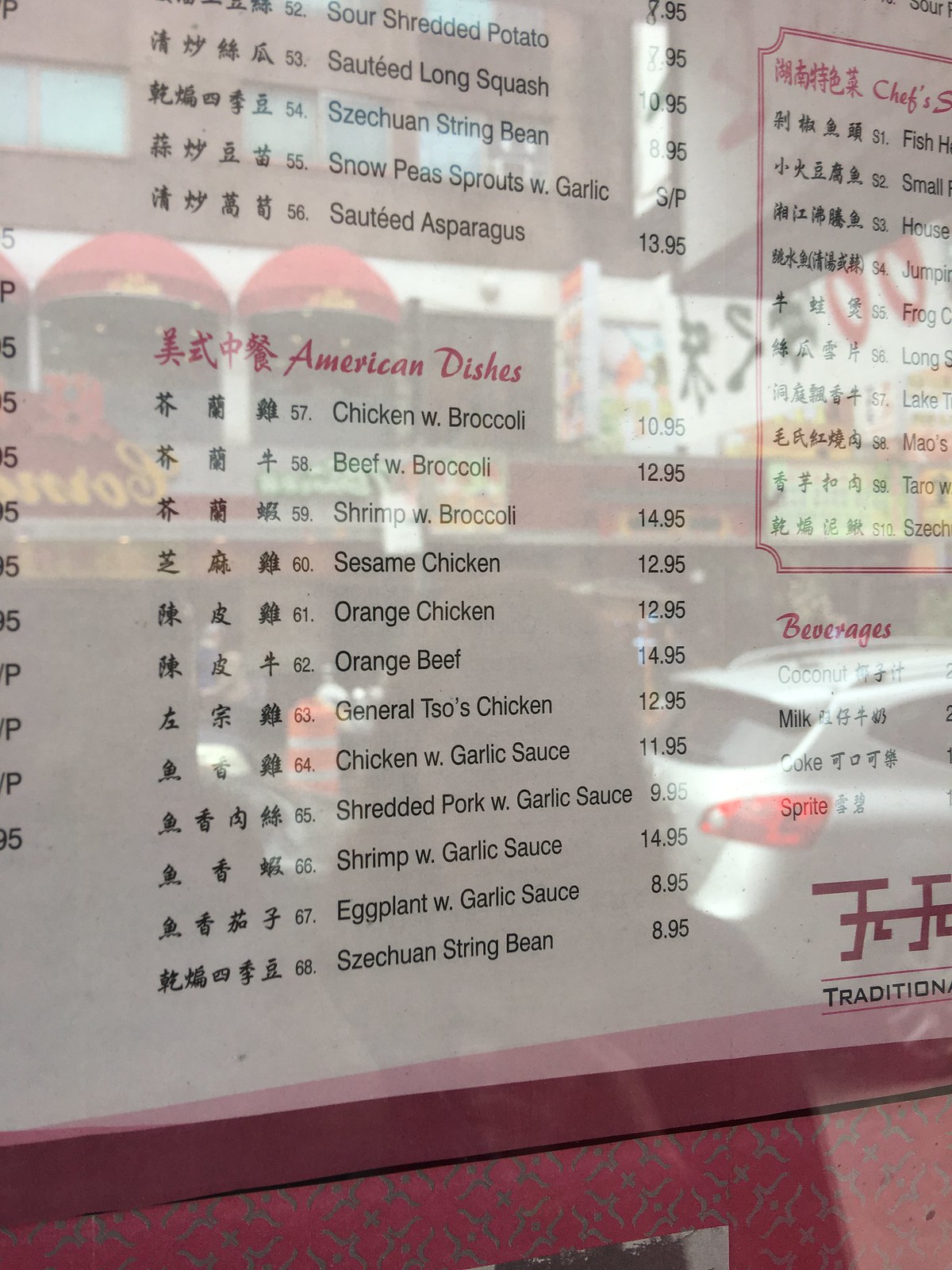Here we have an image of a Chinese restaurant's large menu displayed on a wall adorned with a red and gray pattern reminiscent of a booth's backrest. The menu is encased in glass, reflecting the exterior scene—a streetscape featuring white buildings with red arches and the back end of a white car with red tail lights. The menu itself is extensive, printed in black text on a white background, listing an array of dishes. Under the Chinese cuisine section, items such as sour shredded potato, sautéed long squash, Szechuan string beans, snow peas with sprouts and garlic, and sautéed asparagus are featured. Additionally, an American dishes section is highlighted in red text, including popular items like chicken and broccoli, beef and broccoli, shrimp and broccoli, sesame chicken, orange chicken, orange beef, General Tso's chicken, chicken with garlic sauce, shredded pork with garlic sauce, shrimp with garlic sauce, eggplant with garlic sauce, and Szechuan string beans among numerous other offerings.